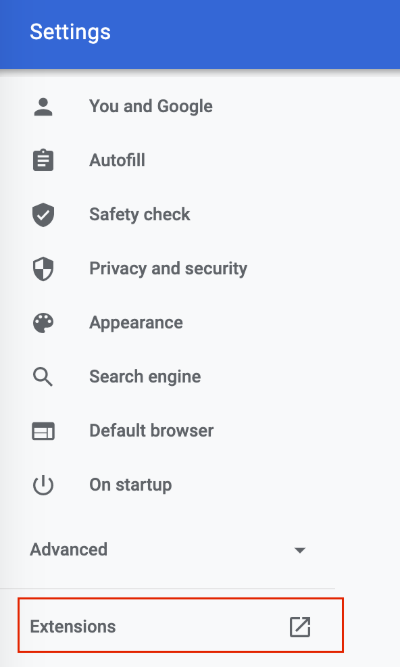The top portion of the image features a long blue rectangle with the word "Settings" spelled out as S-E-T-T-I-N-G-S in the upper left corner. Directly below this, there is an icon of a circle with a person's shoulders, representing a silhouette, next to which are the words "You and Google" in black text. 

Following that, there is an image of a notebook with the word "Autofill" displayed to its right. Below this, a black circle containing a checkmark is labeled as "Safety Check". Progressing downward, a shield symbol with several squares inside is accompanied by the text "Privacy and Security".

Next in line is an icon resembling a wheel, indicative of a cog or gear, with the word "Appearance" situated to its right. Further below, there is a magnifying glass icon with the words "Search Engine" beside it. Continuing downward, an icon representing a square with a long black line across the top is labeled "Default Browser". 

Lastly, there is a nearly filled circle with a small vertical line inside, with the words "On Startup" to its right. Below this is the word "Advanced" accompanied by an arrow pointing downward. The final element is an outlined red rectangle containing the word "Extensions". To the right of this, there is a square icon with an arrow pointing up and to the right.